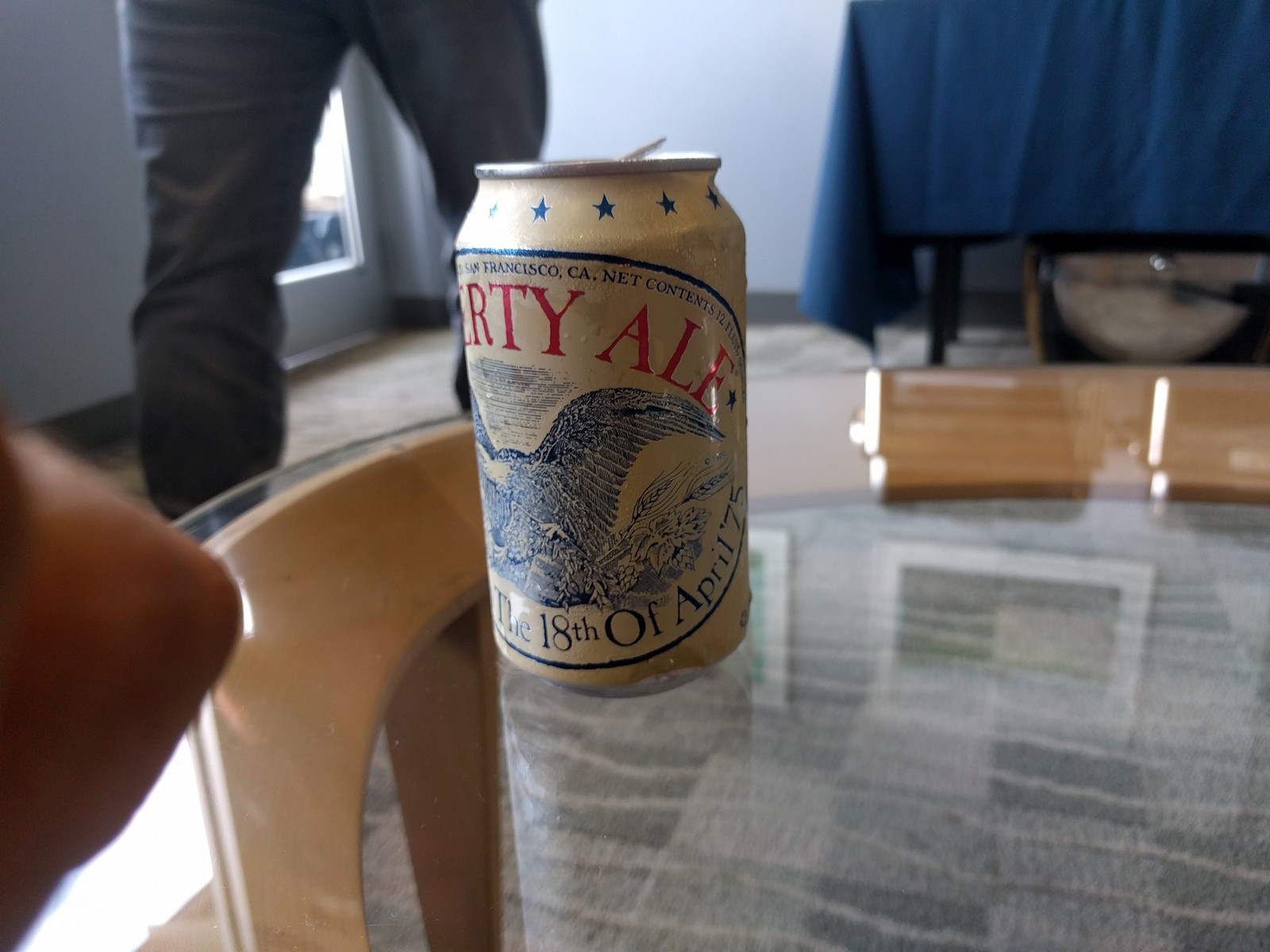In the image, we see a bright, well-lit, modern room with clean, white or gray walls and light beige carpet featuring a wave and checkered design. The central focus is a can of beer or ale resting on a round glass table with light wooden legs. The can is beige with a blue bald eagle graphic and blue stars around the neck. Partially visible text on the can reads "R-T-Y A-L-E," likely indicating "Liberty Ale,” with the phrase “18th of April, 75” curving upwards in blue letters under the eagle. The image appears to be taken from a first-person perspective, as the left hand knuckles of the photographer are visible at the bottom left corner, suggesting the photo was taken with their right hand. In the background, a person wearing denim jeans is seen walking away from the table, with a blue tablecloth-covered table or object slightly visible further back. Between the person's legs, there is a glimpse of a window or a door with light streaming through.